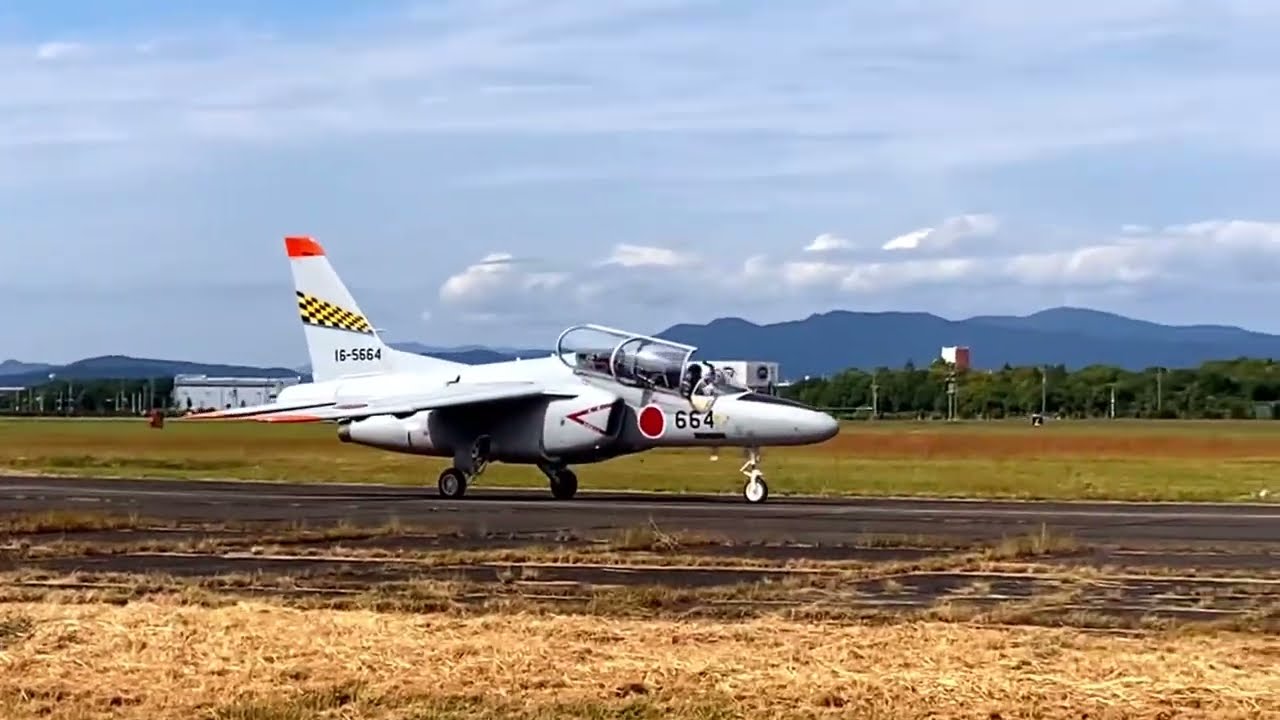The image showcases a striking photograph of a white fighter jet, prominently marking the focal point as it rests on an aging runway. The aircraft, adorned with the number "664" in bold black on its nose, features a notable red circle adjacent to the number, which stands out against its sleek, light gray-blue fuselage. The jet's distinctive tail flaunts a yellow and black checkered emblem and red-tipped fins, alongside a smaller black text "16-5664" towards the back. The wings, partially obscured due to the side angle of the shot, appear to have a gray-blue tint with red tips.

The runway, stretching from the right to the left of the image, appears worn with patches of grass and shrubbery intruding upon the paved surface. In the immediate foreground lies a patch of brown and yellowing grass, adding a touch of contrast to the scene. 

Beyond the runway, a vast green field spreads across the middle of the image. Trees line up in parallel along the horizon, their lush green tops providing a natural border against the backdrop. Further in the distance, power lines are faintly visible, trailing across the landscape towards a majestic mountain range that spans the entire width of the photograph.

Above, the sky is a canvas of mixed weather conditions, showcasing an array of white and gray clouds floating amidst patches of blue, hinting at a clear daytime setting. To the left, a small white building peeks into the frame. The overall composition captures the serene yet commanding presence of the fighter aircraft against a backdrop of natural and man-made elements, culminating in a visually compelling scene.